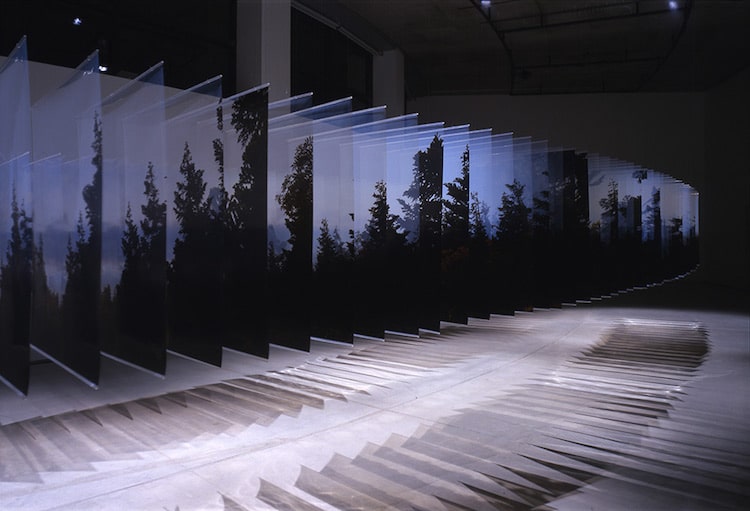The image depicts a striking art installation in an empty warehouse gallery space. The installation consists of numerous glass panels, potentially acrylic, arranged in a row extending indefinitely into the background. Each panel features different silhouettes of trees, creating an effect reminiscent of animation frames when viewed sequentially or from certain angles. The ambiance is dark and moody, with overhead lights illuminating the panels and casting intricate, fan-like shadows across the floor. This interplay of light and shadow enhances the ethereal and reflective quality of the exhibit, transforming the space into a mesmerizing, layered scene of natural silhouettes.